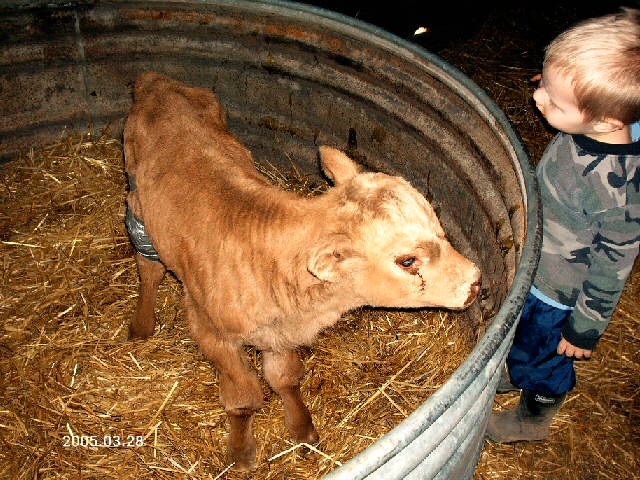In this detailed photograph, a young blonde boy, wearing a green camouflage long-sleeve shirt, dark-colored pants, and dirty black rubber boots, stands next to a large, rusty, round metal container filled with straw or hay. He gazes down intently into the container, which reaches up to his chest. Inside the container stands a calf with brown fur, accented by a white and tan face, and a notable dark brown line running down from one of its black eyes, giving the impression that it has been crying. The calf’s body is dark brown with hints of tan, and its legs are dark brown, with duct tape or some form of silver material wrapped around its right hind leg. A date, “205-03-28,” is stamped in white at the bottom of the photograph, suggesting a specific time and context. The overall setting appears to be a farm, with straw covering the ground and a muted, dark background, hinting that the image might have been taken at night or in a dimly lit area.